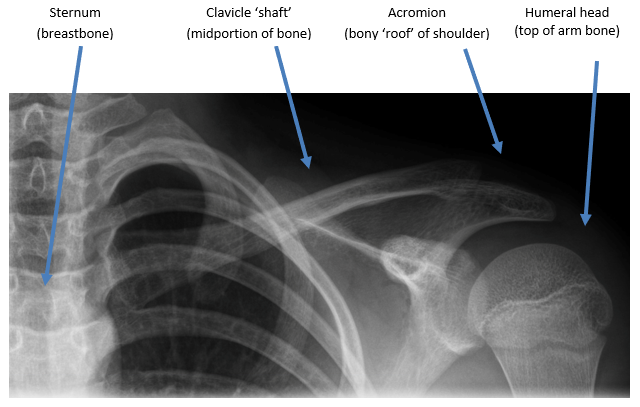This is a detailed black-and-white x-ray image displaying portions of the upper torso, focusing on the left shoulder, ribcage, and spine. The x-ray is mostly in shades of gray, with descriptions pointing out specific skeletal landmarks using fine blue arrows. The labeled parts include the sternum (breastbone), identified by the longest blue arrow, and the clavicle shaft (mid-portion of the clavicle). Further right, the acromion (bony roof of the shoulder) is labeled, followed by the humeral head (top of the arm bone). The image serves as an educational tool, possibly used for medical students or diagnostic purposes to visually map out key anatomical features in this region. The text descriptions are in small black letters, providing clear identification of each highlighted bone and its corresponding region.